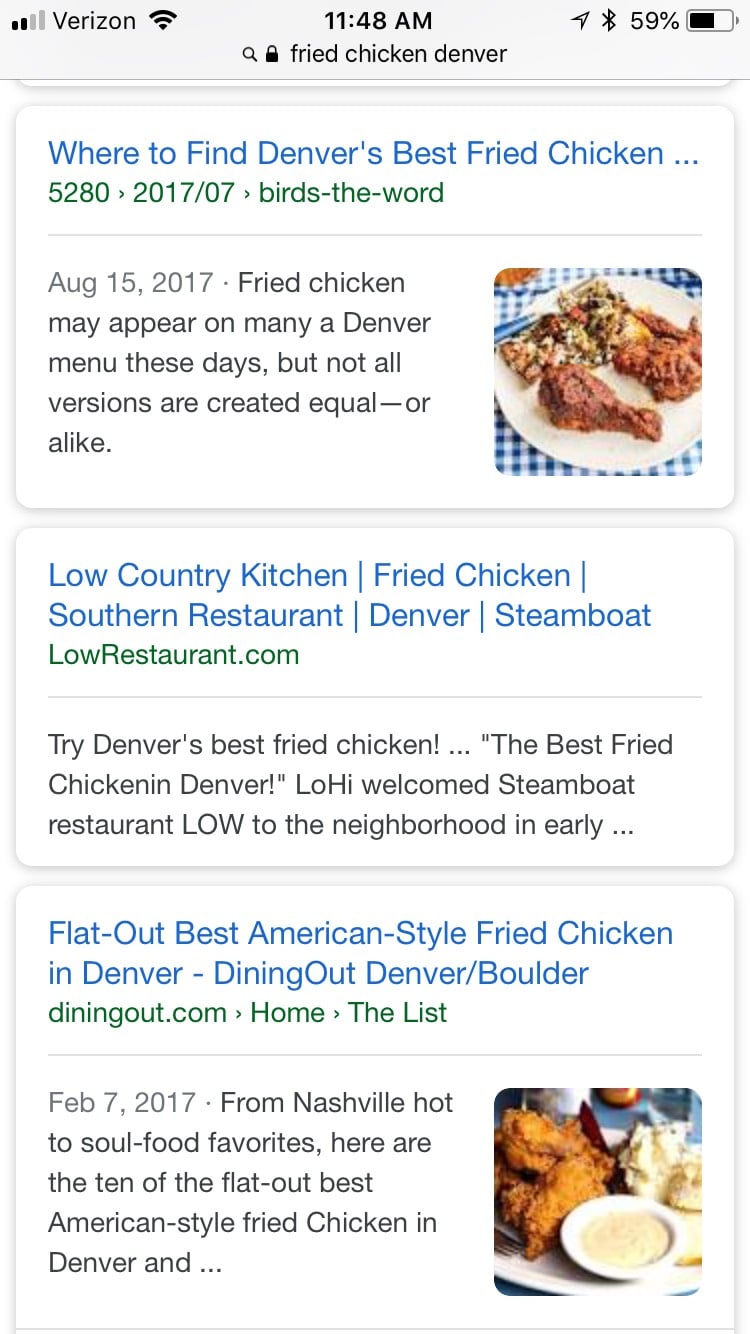The top left corner of the image displays various icons and statuses: two out of four bars for Verizon signal strength, full Wi-Fi connectivity, the time at 11:48 AM, location services, Bluetooth enabled, and a 100% battery charge. The foreground features a close-up of a restaurant setting.

Prominently shown is a glass door with the words "Fried Chicken Denver" etched on it. Below that, a flyer reads "Where to Find Denver's Best Fried Chicken, 5280-2017-707" with an article dated August 15, 2017. The article discusses the varying quality of fried chicken across Denver's menus and mentions specific restaurants known for their exceptional dishes.

On the table, a plate of golden, crispy fried chicken is presented, accompanied by a small ceramic dish filled with sauce. The fried chicken appears perfectly cooked with a crunchy exterior, possibly garnished with herbs or spices. The background shows other dining elements, including blue ceramic containers, further enhancing the overall dining atmosphere.

The caption highlights Denver's notable fried chicken spots: Low Country Kitchen, a southern-style restaurant in Denver, and Steamboat, a neighborhood favorite. The text also references reviews and lists from credible sources such as diningoutdenver.com, which recommend the top ten American-style fried chicken spots in Denver from Nashville hot to soul food favorites.